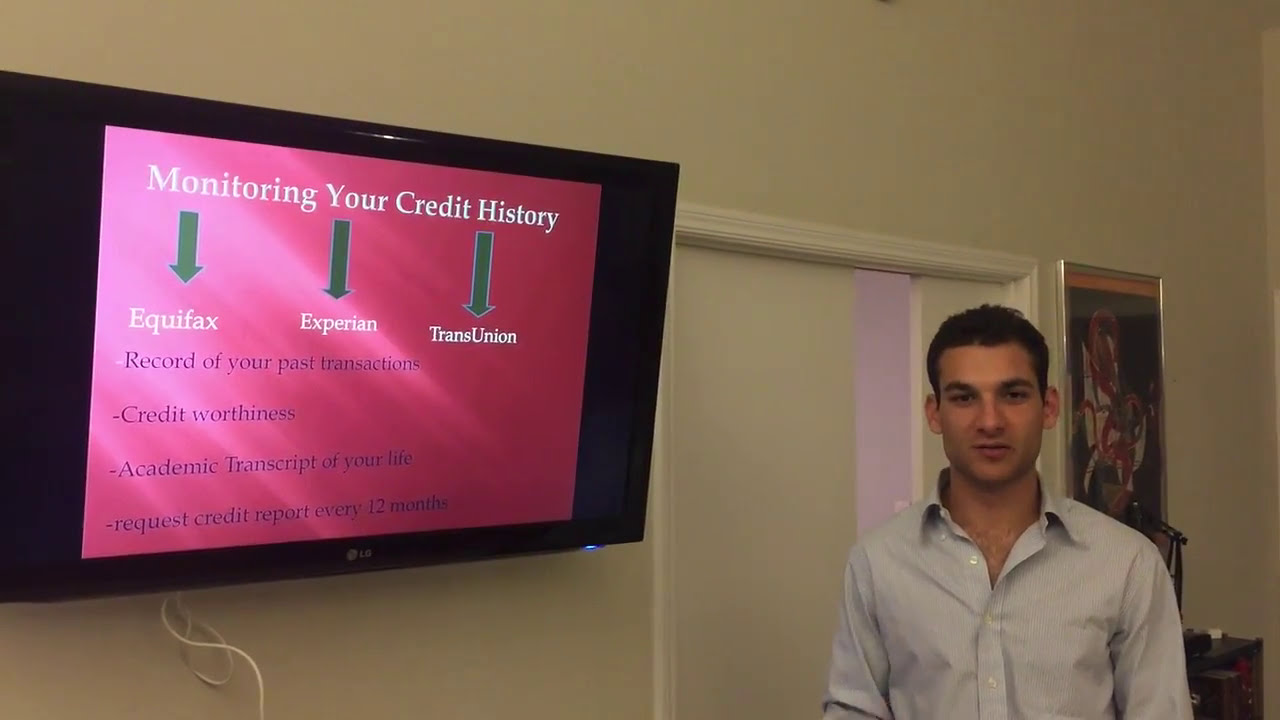The indoor setting appears to be either an office or a home, where a young, olive-skinned man with black hair, dressed in a light blue, possibly striped dress shirt, is standing on the bottom right side of the image. He is looking directly into the camera. On the left side of the image, there is a black flat-screen LG TV mounted on the wall displaying a slide related to credit monitoring. The slide features green arrows pointing to the names of the three credit agencies: Equifax, Experian, and TransUnion. The text on the TV reads, "Monitoring your credit history," and includes points such as "record of your past transactions," "credit worthiness," "academic transcript of your life," and "request credit report every 12 months." The colors in the image include shades of tan, black, pink, purple, green, white, and light blue. This scene seems to depict an educational session or presentation about credit.